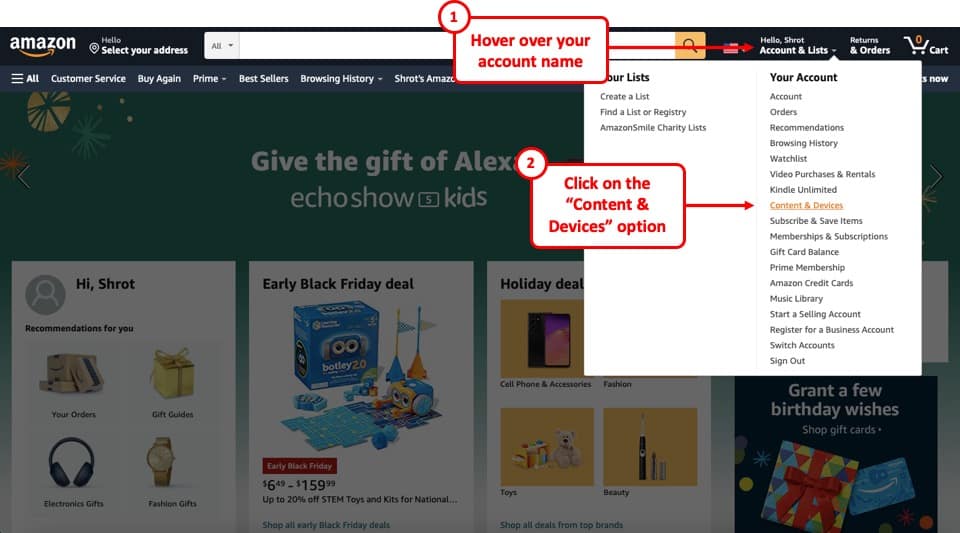This screenshot captures the Amazon website's homepage during a special promotional period. In the upper left corner, the iconic Amazon logo is prominently displayed, featuring the recognizable orange arrow underneath bold white block text. To its right, the text reads "Hello, select your address," followed by a white search bar that's centrally positioned for ease of product searches.

In the section below the search bar, a white box greets the user with "Hi Schrott, recommendations for you." This box contains various icons linked to personalized recommendations. The first icon represents "Your Orders," illustrated by an assortment of Amazon boxes. Next to it, the "Gift Guides" icon showcases a gold-wrapped gift, enticing shoppers with curated suggestions.

Further down on the left side, a category for "Electronic Gifts" is depicted through an image of sleek black headphones. Adjacent to this, the "Fashion Gifts" category features a sophisticated gold watch. To the right, a separate box stands out with bold black text announcing an "Early Black Friday Deal." This box also includes a smaller red box with text emphasizing "Early Black Friday," followed by the price range "$6.49 to $159.99" and an enticing offer of "up to 20% off STEM toys and kits." Beneath this promotional offer, small blue text encourages users to "shop all early Black Friday deals."

The overall layout of this screenshot effectively directs the user’s attention to various shopping categories and special offers, making it a dynamic and engaging preview of the Amazon online shopping experience.